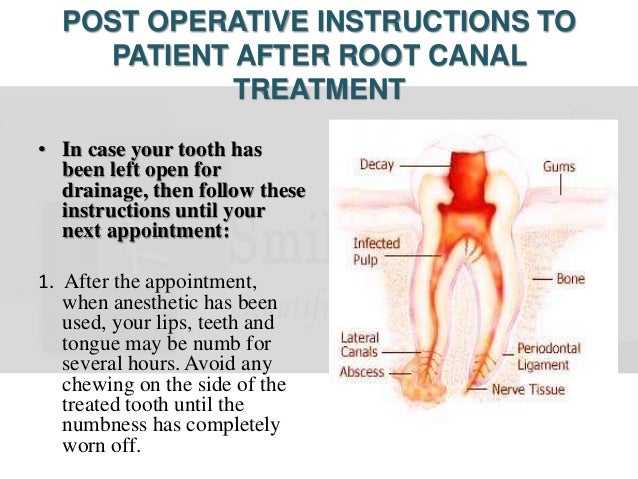The image provides detailed post-operative instructions following a root canal treatment. At the top, in blue font on a white background, it reads "Post-operative instructions to patient after root canal treatment." Below that, in black text, the instructions specify: "In case your tooth has been left open for drainage, follow these instructions until your next appointment. 1. After the appointment, when anesthetic has been used, your lips, teeth, and tongue may be numb for several hours. Avoid any chewing on the side of the treated tooth until the numbness has completely worn off."

To the right of the text, there is an anatomical illustration of a tooth labeled with various parts. The labels indicate "decay" at the top, "gums" at the upper right corner, "infected pulp" in the middle, "bone" and "lateral canals" in the center, "abscess" at the lower left, "periodontal ligament," and "nerve tissue" at the bottom. The image is set against a white background and is oriented upright, displaying a cross-sectional view of the tooth with detailed annotations for each part.